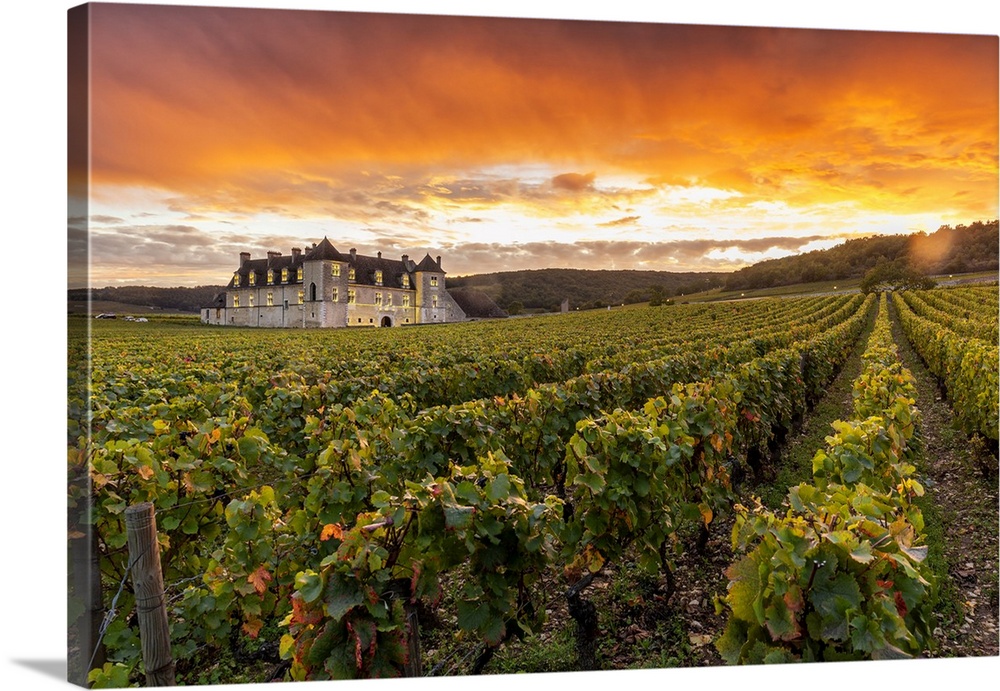This is a captivating photograph mounted on a rectangular board, depicting a vast and meticulously maintained vineyard stretching across the landscape. The camera angle is close to the ground, emphasizing the endless rows of verdant green plants with vine-like leaves, suggesting they might be grapevines. These plants are neatly aligned, showcasing the careful farming practices that maintain the vineyard. In the foreground, a grand, three-story estate with white walls and a brown roof stands prominently to the left. This sizable mansion, possibly with 20 rooms, suggests prosperity, likely derived from the vineyard's produce. Behind the house, small hills rise gently, adding depth to the scene. The sky above is a dramatic display of colors during sunset, with vibrant oranges and reds high above, gradually transitioning to a light blue as it approaches the horizon. A bank of grey clouds rests just above the hills, completing the picturesque view.